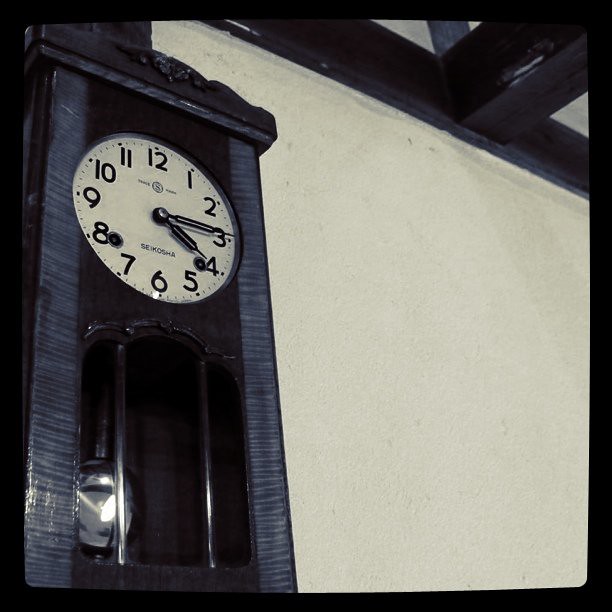This black-and-white photograph captures a detailed image of a grandmother clock mounted on an off-white wall inside a building with visible black wooden beams intersecting across the ceiling. Dominating the left side of the image, the clock's dark brown wooden structure appears in various shades of gray due to the monochrome palette, giving it an interesting graphite gray and slight blue tint. The clock, approximately two and a half to three feet tall, features a glass front showcasing its swinging pendulum, currently positioned to the far left of the image.

Above the pendulum, the white clock face is clearly visible, marked with standard black numbers from 1 to 12 and bold black hands indicating a time of about 4:15. The top of the clock is adorned with an ornate, scalloped wood covering, adding a touch of elegance to its simple yet classic design. Though a brand name or text is somewhat obscured, a label reading "S-E-K-H-O-H-A" is faintly visible above the 6 o'clock position.

The surrounding architecture, with its dark beams and the faint outline of a wooden plank in the upper right corner, contrasts against the lighter wall, framing the clock and highlighting its antique charm and stately presence within the room.